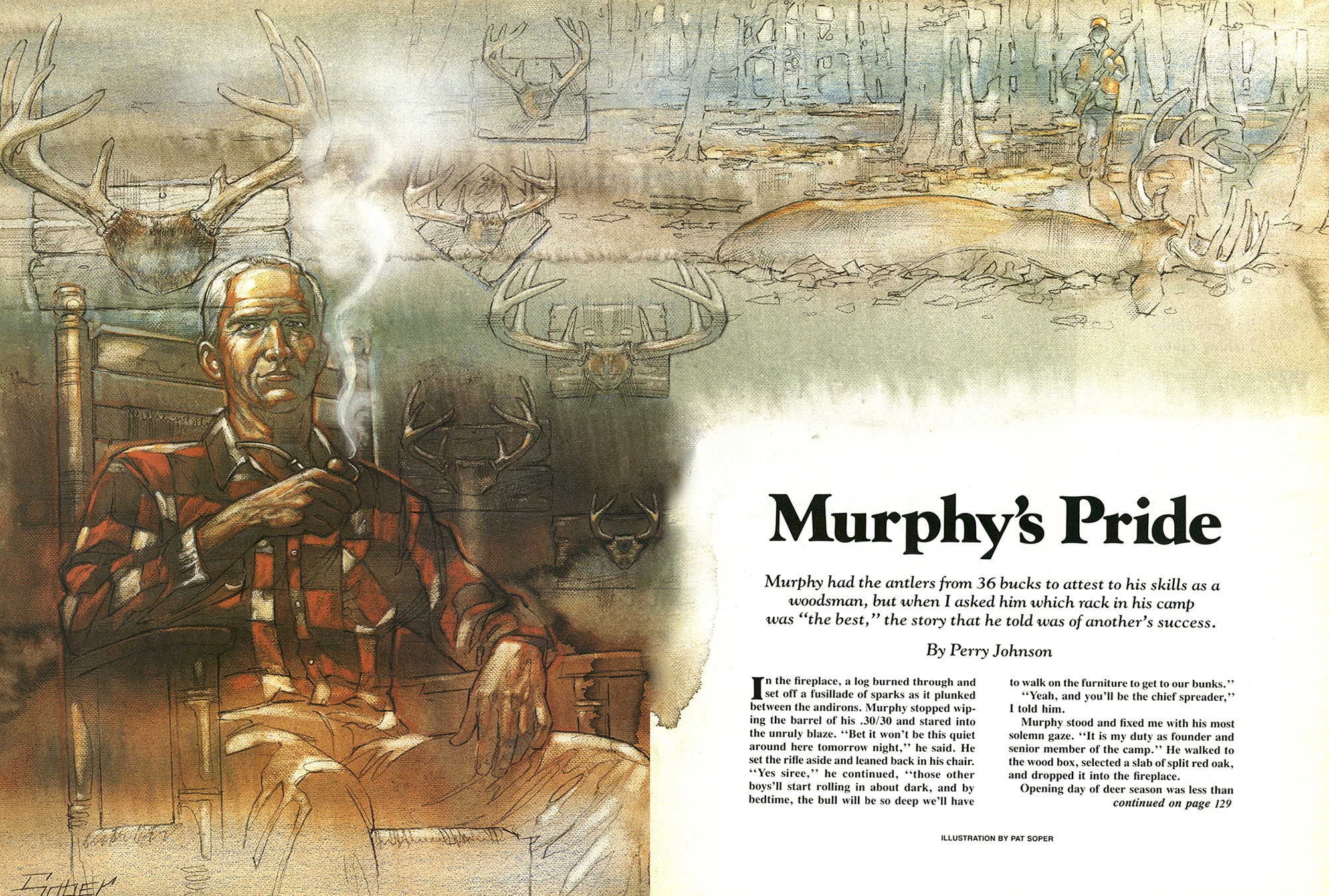The image is a detailed poster for a short story titled "Murphy's Pride" by Perry Johnson. The main illustration features a balding man in his 50s, wearing a red, white, and dark burgundy flannel shirt and white khaki pants, sitting in a high-backed rocking chair while smoking a pipe, with visible smoke curls. Surrounding him on the walls are mounted deer antlers, trophies from his hunting expeditions displaying his skills as a woodsman. The bottom left of the poster includes a caption stating, "Murphy had the antlers from 36 bucks to attest to his skills as a woodsman, but when I asked him which rack in his camp was the best, the story that he told was of another success by Perry Johnson." In the background, there’s a second drawing of a hunter in full camouflage and an orange cap, holding a rifle next to a freshly shot stag, suggesting a reflective or nostalgic moment. The poster's bottom left is signed, tying it all together as an introduction to the story.